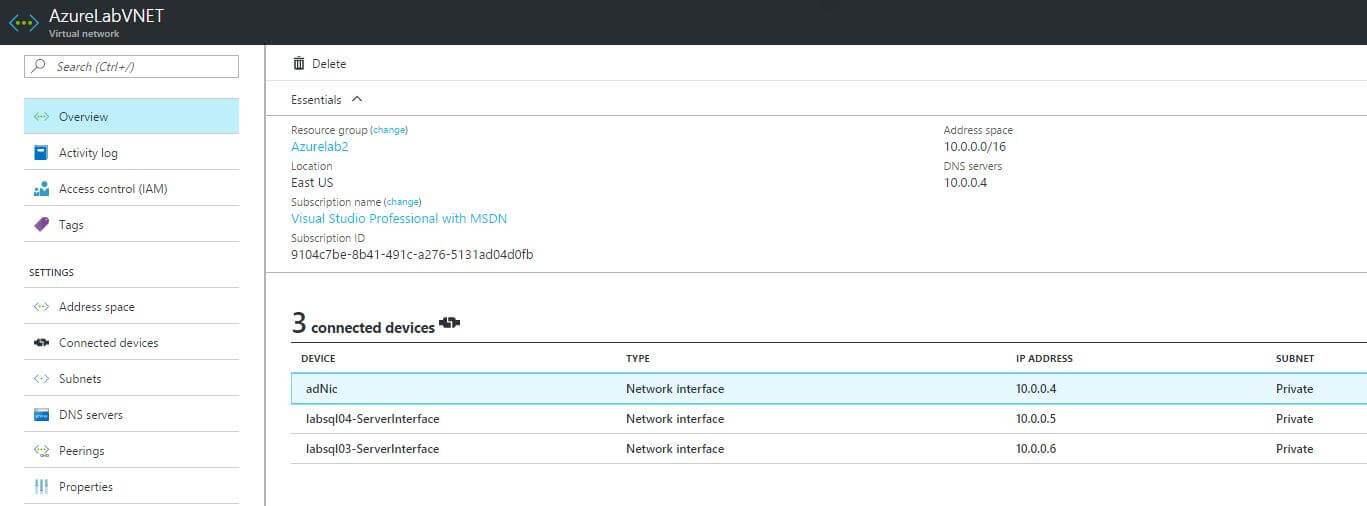The image features a user interface for a network management tool. At the very top of the interface, there is a long black bar with "azurel.ab" and "VNFT" prominently displayed in capital letters. Directly below this black bar is a search bar positioned to the left, next to a blue rectangle labeled "Overview."

Beneath the "Overview" section, there are several categorized options listed vertically: "Activity Log," "Access Control," "Tags," "Settings," "Address Space," "Connected Devices," "Subnets," and "Properties." To the far right of these categories is a clickable option labeled "Delete," with another subcategory just below it.

The interface indicates that the current location is "East US." In the address space section, the specified range is "100-15." The connected devices category lists "three connected devices." One device is highlighted in a blue rectangle, showing detailed information: the device is "ANIC," its type is "Network Interface," it has an IP address of "10.0.0.4," and it is marked as "Private."